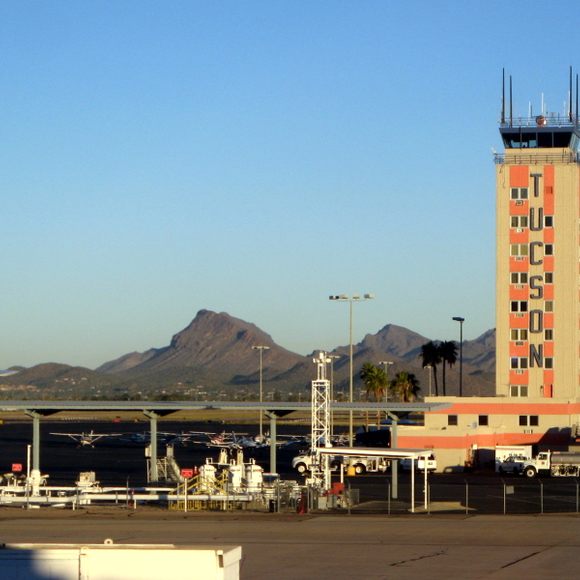This detailed outdoor image captures the Tucson Airport in Arizona under a clear blue sky, with no clouds in sight. The airport features prominently with a distinctive watchtower, a tall, narrow structure adorned with numerous control tower-type windows and large antennas on top, rising on the right side of the frame. Clearly labeled with "TUCSON" in large letters, the building has a peach-colored facade with orange accents. Below the tower, there are various service vehicles, including large trucks and water trucks. Small airplanes, parked under canopies, can be seen in the middle ground. In the background, there's a low mountain range with sparse vegetation, dominated by gray dirt, and the distant city nestled at the mountain's base. Tall light poles are scattered throughout the airport area, and the foreground showcases an open expanse of tarmac dotted with service vehicles, casting long shadows in what seems to be the late afternoon sun.